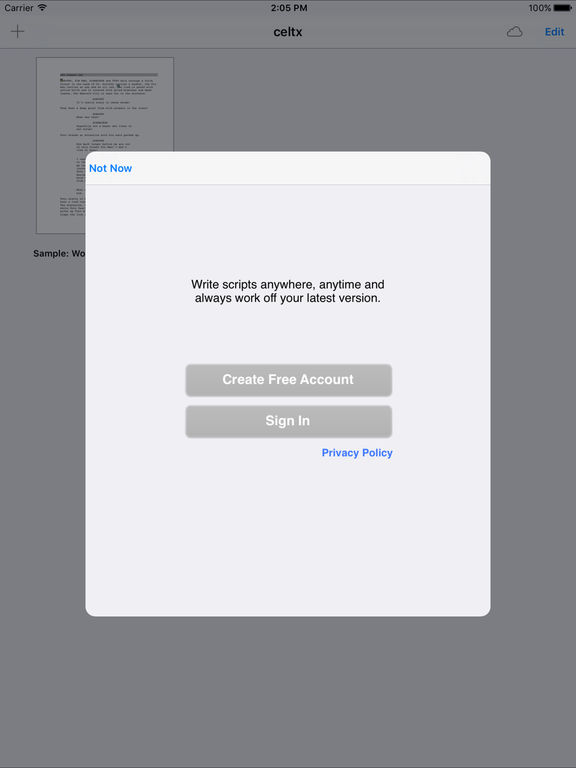The image showcases a screenshot of a vertically-oriented web page with a translucent gray overlay that casts a shadow over the underlying content. At the center of the image, there is a prominent white, rounded-corner pop-up box. In the upper left-hand corner of this pop-up, blue text reads "Not Now." The main message in the center of the box promotes a scriptwriting feature with the text: "Write scripts anywhere, anytime, and always work off your latest version."

Below this message, there are two light gray buttons. The upper button contains the white text "Create free account," while the lower button says "Sign in." At the bottom of the pop-up box, blue text states: "Privacy policy."

Visible in the backdrop of the image, the upper left corner of the web page displays the word "Carrier." The center of the header indicates the time, "2:05 PM," while the upper right corner shows the battery status at "100%." Directly beneath the time is the text "C-E-L-T-X," accompanied by a plus icon, a cloud icon, and an edit button. An illegible sheet of text and the word "Sample" are faintly visible behind the top left-hand corner of the pop-up box.

This detailed depiction captures the overlay and informational elements of the web page interface clearly, emphasizing the focus on user interaction and account creation options.